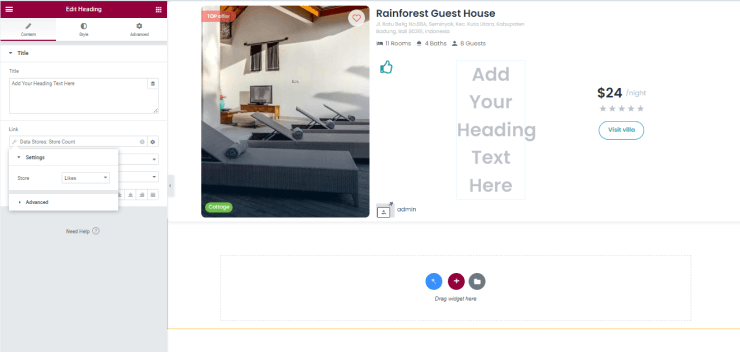Screenshot of Website Template for Rainforest Resort:

The image showcases a website template under construction. On the left side, there is a designated title field or section, followed by a sizeable text box meant for a description or other important details. Centrally placed within the template is a photograph depicting several lounge chairs, typical of those found at a resort poolside, suggesting a luxurious and relaxing ambiance.

In the upper right corner, the header reads "Rainforest Guesthouse" in prominent text. Below this, there is an address displayed in a faint grey font, making it barely legible. Further details specify that the guesthouse features 11 rooms, 4 bathrooms, and can accommodate up to 8 guests.

In the middle part of the template, there is placeholder text that reads "Add your heading text here," indicating where the main title or headline will eventually appear.

To the right, the nightly rate is stated as "$24," with a row of five empty stars below it, likely representing a rating system. Beneath this, a clickable button is labeled "Visit Villa," inviting visitors to proceed with booking or viewing more detailed information.